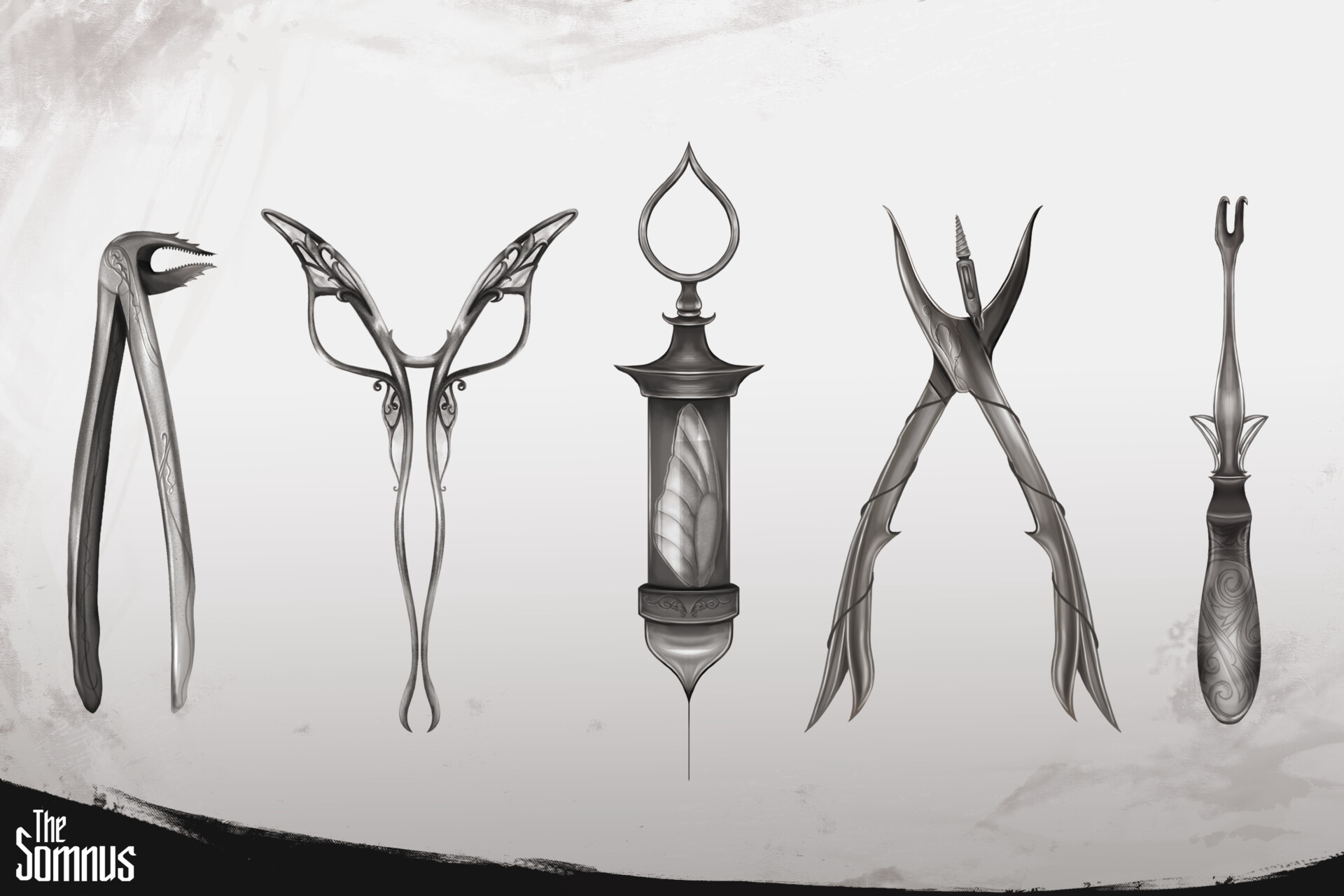The hand-drawn illustration, set against a white background with gray splotches reminiscent of distressed or used paper, features five distinct, detailed metal instruments. Each tool, rendered in either pencil or colored pencil, is depicted in shades of gray and black. There’s an underlying black ink curve across the bottom of the image, with the words "The Somnus" inscribed in a stylized font in the left-hand corner.

From left to right, the instruments include:

1. A unique pair of tweezers, featuring a smaller pair of tweezers at the end.
2. Tweezers with a design that mimics butterfly wings.
3. A syringe with a very sharp needle, housing what appears to be an artistic rendition of a butterfly wing.
4. A pair of pliers that also incorporates a drill-like element.
5. A long, hook-like tool.

These instruments combine elements of traditional tools with whimsical, almost surreal insect-inspired designs, blurring the line between functionality and fantasy.